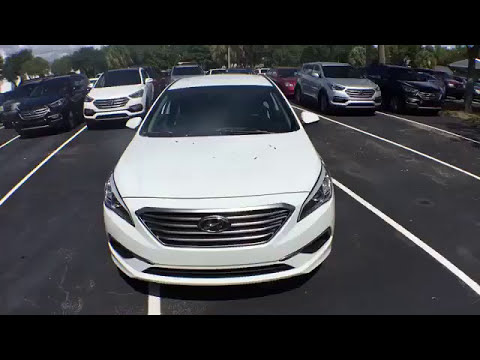This full-color landscape photograph, bordered by black stripes on the top and bottom, captures a parking lot scene during the daytime. The central focus is a white car, possibly a Hyundai, which is parked crookedly, partially encroaching into an adjacent space and disrupting the alignment. Surrounding this vehicle, a variety of other cars—including white, black, silver, and red—are parked properly, all facing the camera. The background features a dense tree line and a sky filled with clouds, adding a natural contrast to the orderly rows of cars. The image lacks the presence of people, emphasizing the stillness and the slightly chaotic parking of the leading sedan in an otherwise orderly setting.